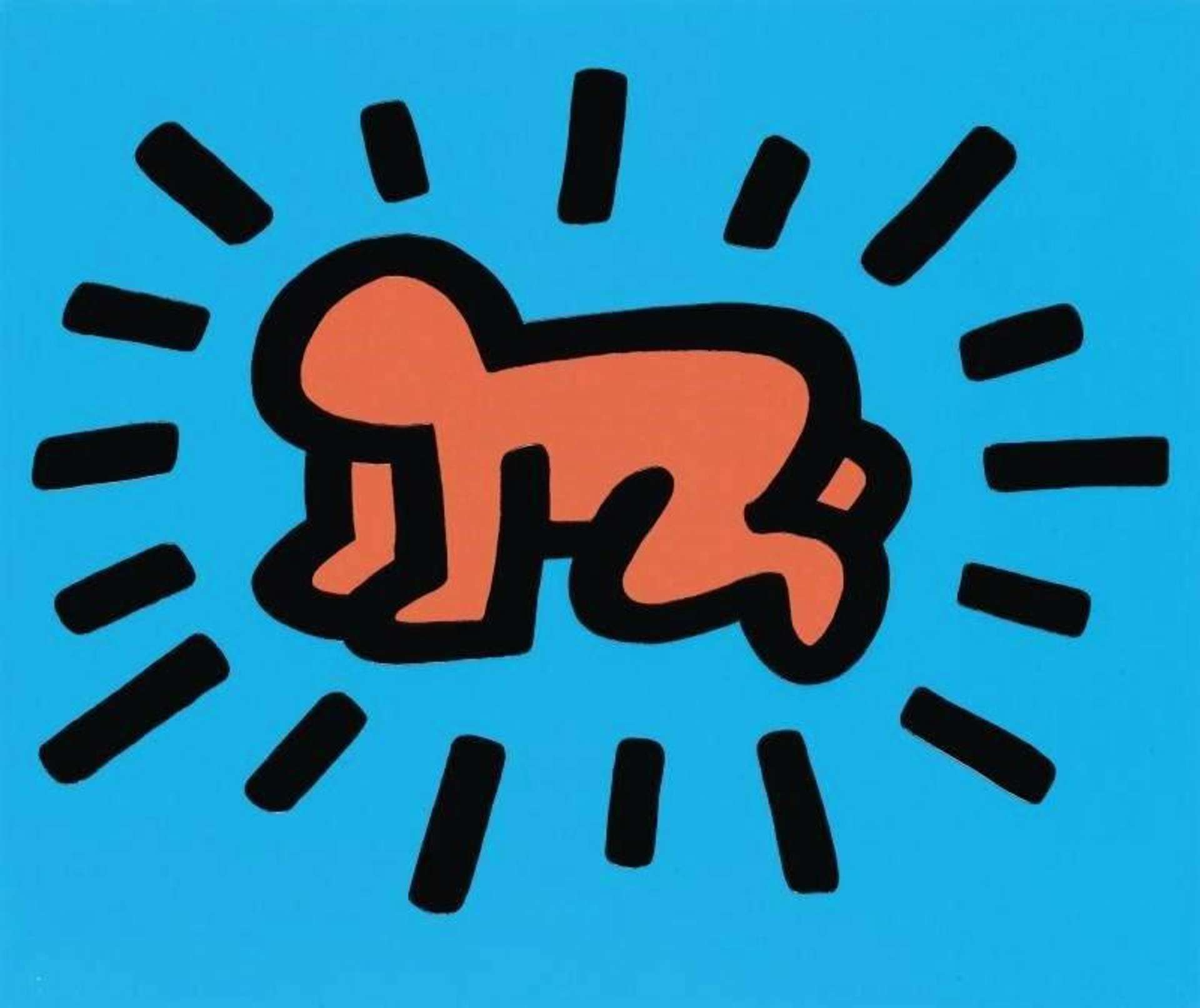The image is a simplistic cartoon graphic with a light blue background, depicting a human figure on its hands and knees. The figure is outlined with thick black lines and filled with an orange-red color, devoid of any facial features or details. Surrounding the central figure are various black lines radiating outward, some longer and some shorter, resembling the rays of a sun. These lines, similar in thickness to the outline of the figure, suggest a sense of energy emanating from the person. This iconographic image, reminiscent of designs seen on t-shirts, is characterized by its stark, minimalistic style and repetitive line pattern.